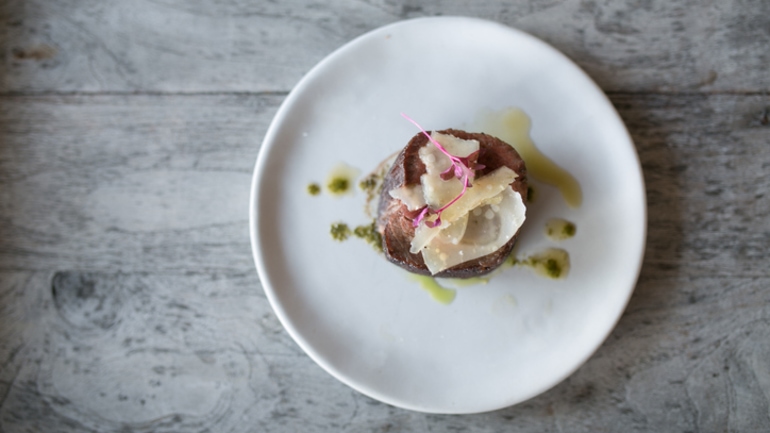A meticulously presented delicacy rests on a basic white, perfectly circular plate set against a grey wooden tabletop with visible grain details. The centerpiece of the meal appears to be a small cut of beef, possibly filet mignon, encircled by a drizzle of a light, green-hued sauce, potentially cream-based. The steak is adorned with large curls of fresh white cheese and a striking pink garnish, which could be a vibrant flower or even pink cabbage. The presentation resembles the elegant, artistic plating typical of high-end fictional restaurants, emphasizing both visual appeal and culinary precision.